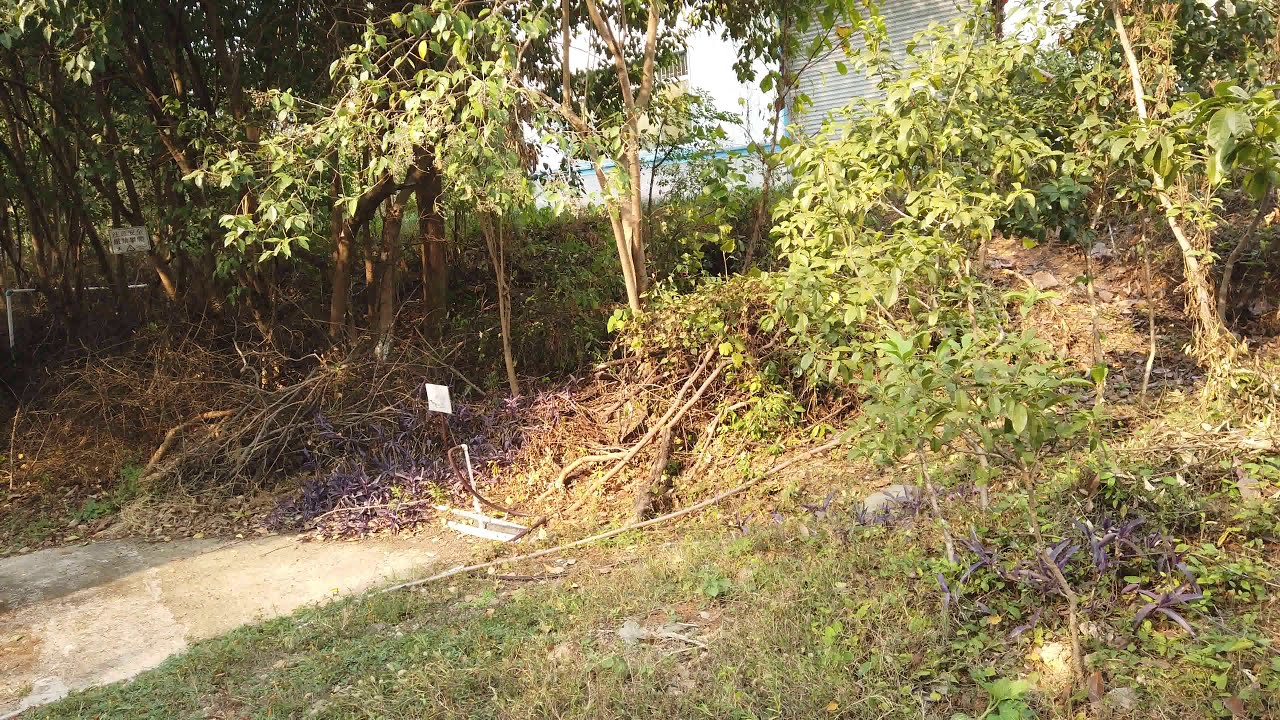The image depicts a neglected grassy area situated behind a house, characterized by its overgrown state and scattered debris. A narrow cement pad is visible amid the tall, unkempt grass. The scene suggests it might have once been a cared-for space since there are remnants of deliberate plantings, like distinct purple grasses often used to border flower beds. At the bottom left corner, a pathway begins, leading diagonally up towards the center. This path is surrounded by twigs, brush, and leaves. A small white sign stands somewhat indistinctly amidst this clutter. Beyond the pathway, clusters of small trees with narrow trunks and brown roots are visible, providing ample shade. The area is dotted with more bushes and broken branches. A fence runs behind the trees, its light blue top hinting at an expanse beyond. Behind the fence, a gray-brick wall stretches across the background, over which patches of light blue sky peek through the foliage. The sun bathes the leaves in light, although it remains out of the frame.